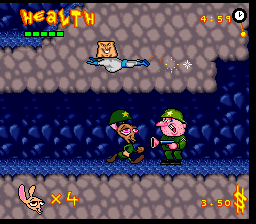The image is a detailed screenshot from a Ren and Stimpy-themed video game, which appears to be a side-scrolling adventure set in a tunnel. The game mechanics allow characters to move horizontally from left to right, with the story progressing in that direction. In the upper left-hand corner of the screen, the word "Health" is prominently displayed in yellow lettering, accompanied by five green bars that indicate the character's current health status. 

On the upper right-hand corner, also in yellow lettering, the numbers "459" are shown next to a small clock icon, likely representing the remaining time for the level. The lower right-hand corner displays the amount "$3.50" in yellow font, indicating the character's collected money. In the lower left-hand corner, there's an icon of a character's head, possibly Ren or Stimpy, with "x4" next to it, suggesting the number of lives remaining.

The scene itself features two characters dressed in green army uniforms complete with matching helmets. One character resembles a kangaroo, while the other could either be a pig or a pink-skinned human. Adding a whimsical touch to the scene, a superhero with a head resembling a piece of toast is seen flying above them.